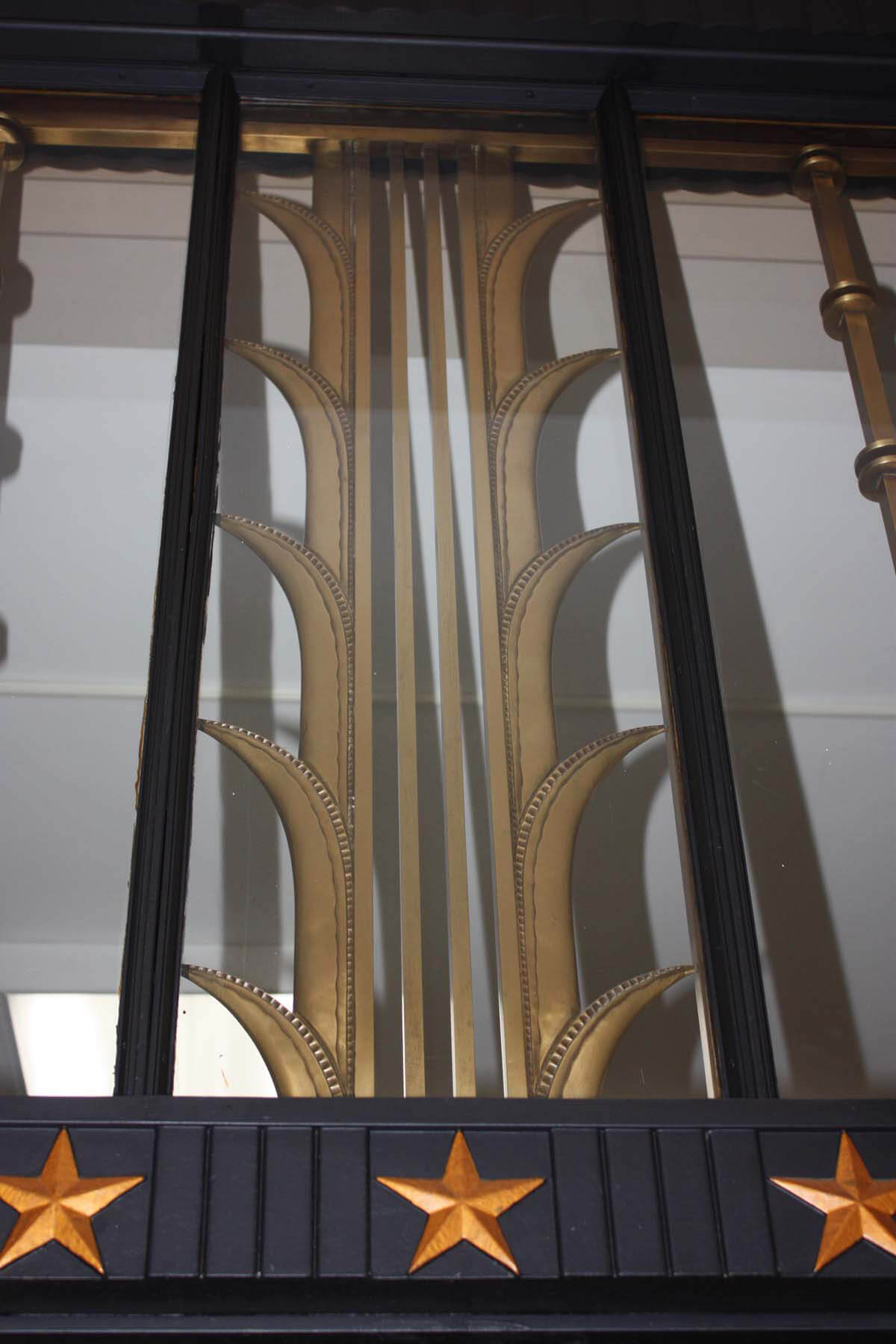The image is a photograph capturing an ornate section of a building's window, likely situated high towards the roof. The window features a distinctive black band running along its bottom edge, adorned with three evenly spaced, golden five-pointed stars. Each star displays a rich hue, described by some as coppery or mustard-colored, adding a touch of elegance. Above these stars, the central section of the window is framed by two vertical black separators. In the middle of this section, a gold multi-line decoration rises vertically, reminiscent of delicate gold leaf work. This decoration includes ornate, branch-like extensions with five points on either side, curving outward much like the blades of swords, and adorned with dotted details along the top and tips. Behind this elaborate design, the glass reveals a backdrop of closed white blinds, further enhancing the window's intricate appearance against the contrasting interior. The surrounding structure appears to be built with mahogany-colored wood, contributing to the overall sophisticated and classic aesthetic.